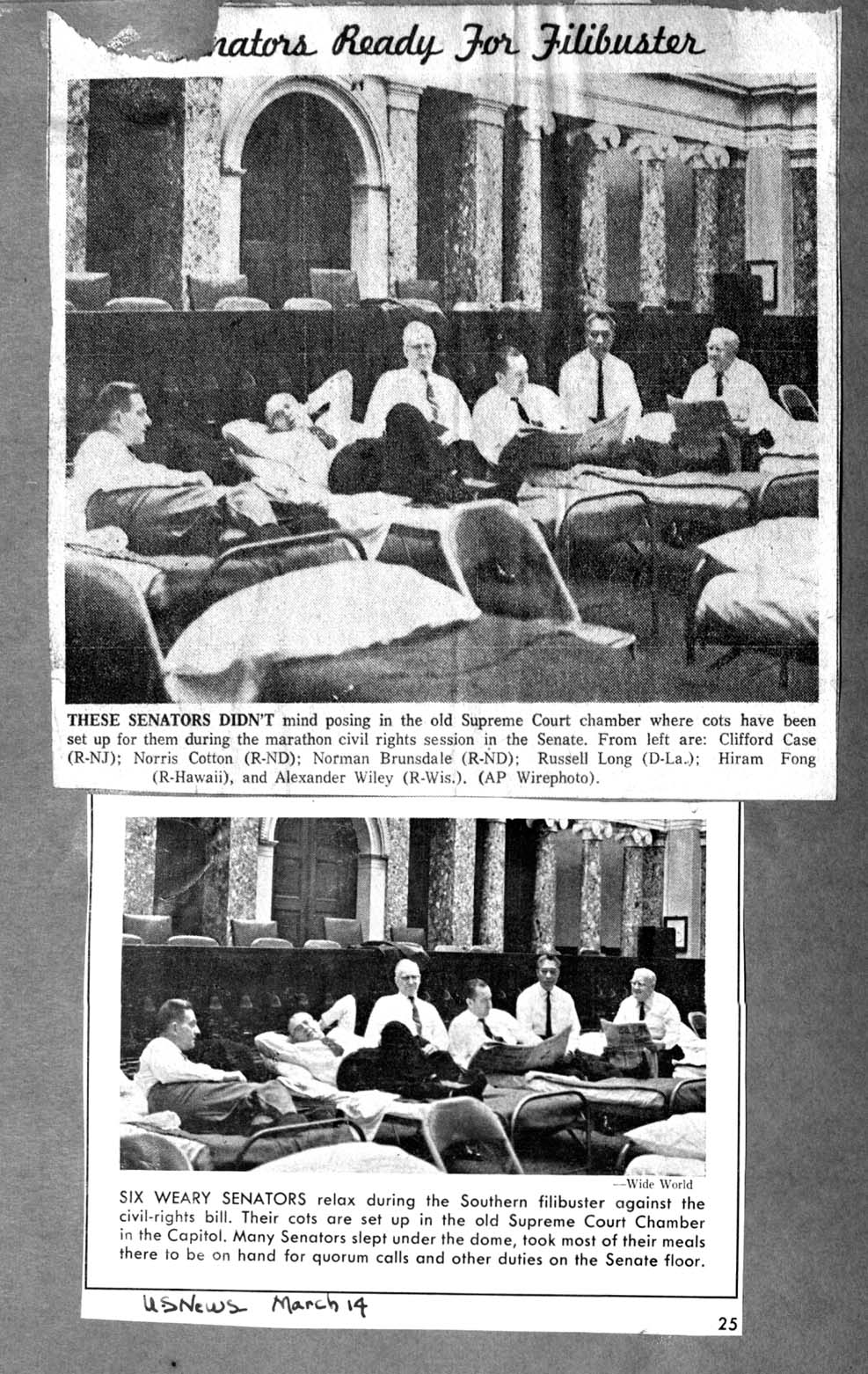The image features two vertically-aligned black-and-white newspaper clippings against a dark gray board background. The top clipping, occupying the upper half of the board, shows six older white men in white button-down shirts, ties, and pants, reclining on cots set up in the old Supreme Court chamber. These men are U.S. senators: Clifford Case (Republican, New Jersey), Norris Cotton (Republican, New Hampshire), Norman Brunsdale (Republican, North Dakota), Russell Long (Democrat, Louisiana), Hiram Fong (Republican, Hawaii), and Alexander Wiley (Republican, Wisconsin). The caption below this photo reads, "These senators didn't mind posing in the old Supreme Court chamber where cots were set up for them during the marathon civil rights session in the Senate."

The bottom clipping, smaller and also in a vertical rectangle, is a secondary description of the same image. It states, "Six weary senators relaxed during the Southern filibuster against the civil rights bill. Their cots are set up in the old Supreme Court chamber in the Capitol. Many senators slept under the dome, took most of their meals there to be on hand for quorum calls and other duties on the Senate floor." This photo was published in U.S. News on March 14th.